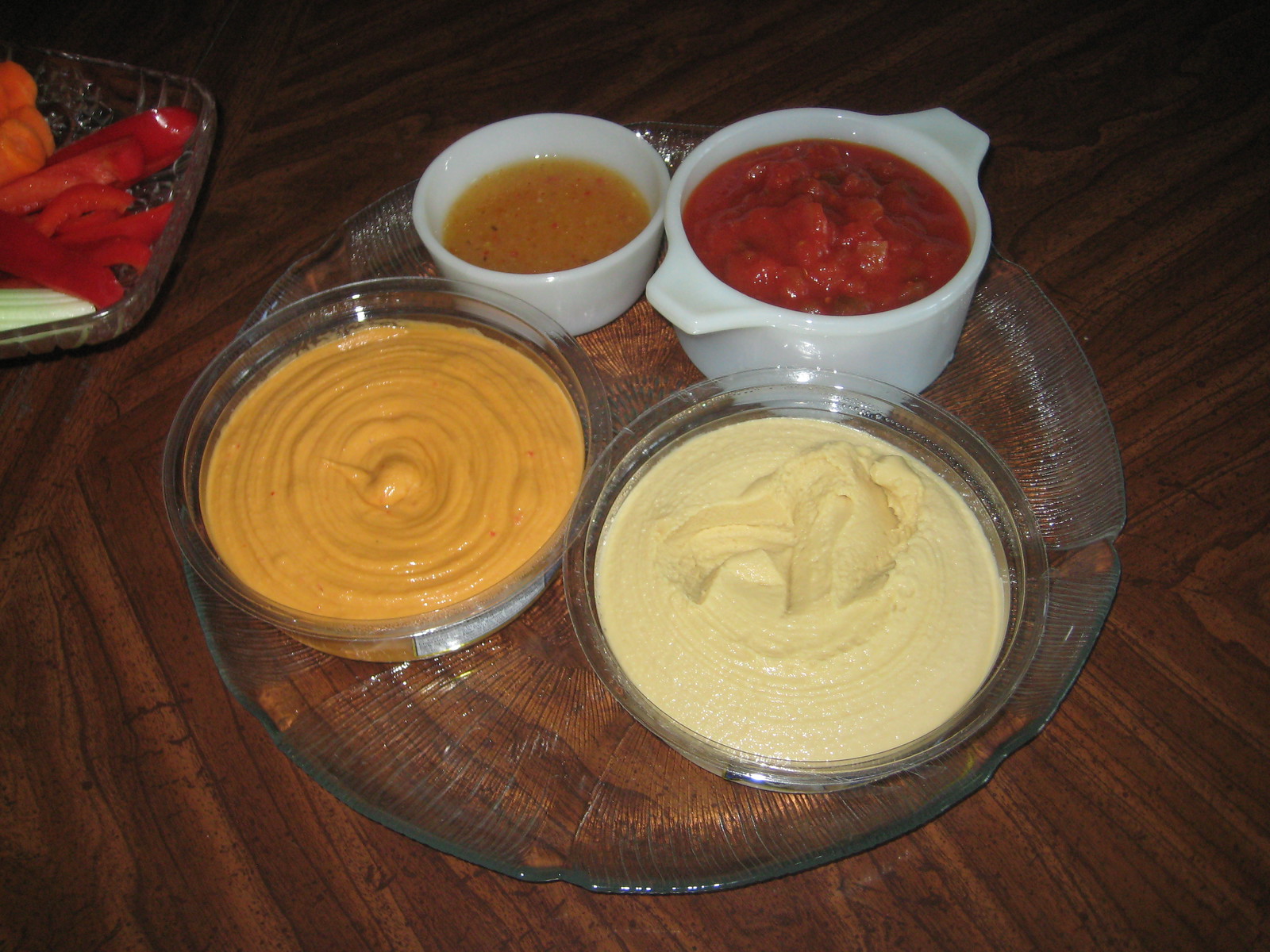The image is a detailed color photograph taken from above, showcasing a meticulously arranged assortment of food items on a dark wood table. Central to the composition is an intricately designed circular glass dish with subtle ribbing running from its center to the edges, and uneven contours around its circumference. Nestled within this dish are two smaller glass bowls—one filled with an orange dip, the other a pale yellow dip showing signs of use. 

In the background, there are two white ceramic bowls: a smaller one to the left holding an orange dip flecked with black spices, and a larger bowl with handles to the right containing a chunky red mixture, possibly pureed strawberries. Additionally, in the upper left corner of the frame, there is a squarish glass tray with assorted cut vegetables, including peppers, carrots, and celery, intended for dipping. The entire arrangement is artfully placed on the richly stained dark wood table, creating a visually appealing tableau of dips and accompaniments.